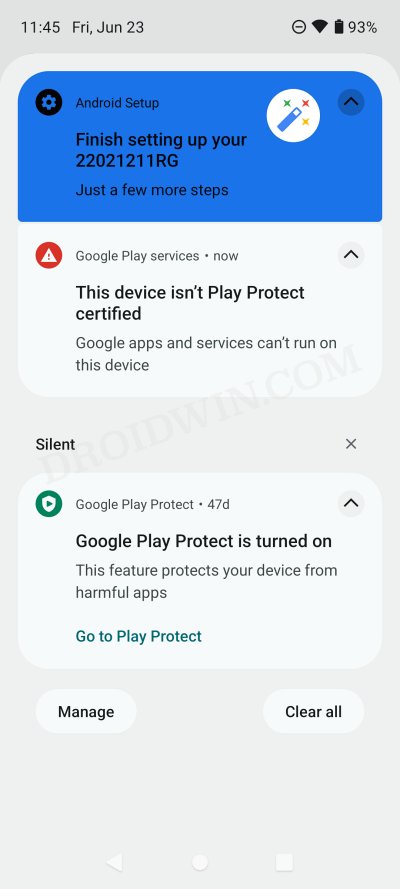This is a screenshot from a cell phone taken on Friday, June 23rd, at 11:45 AM. The top of the screen displays the current time along with icons indicating a Wi-Fi connection and a battery level at 93%. The upper portion of the screen, set against a blue background, shows a notification titled "Android Setup" with the instruction to "Finish setting up your 22021211RG" and mentions that there are just a few more steps to complete. To the left of this text is a gear icon, and to the right is a white circle containing an icon of a magic wand with sparkles.

Below this section, the background is white and contains a message stating, "Google Play services now." It warns that the device isn't Play Protect certified and that Google apps and services can't run on this device. Next to this message is a red circle with a white triangle and an exclamation point in the center.

Further down, another message indicates "Silent. Google Play Protect 47 days." It notes that Google Play Protect is turned on and explains that this feature protects the device from harmful apps. There is an option to go to Play Protect, accompanied by a green icon with a white shield in the center.

At the bottom of the screen, there are options labeled "Manage" and "Clear All," each housed within white oblong shapes. A watermark diagonally spans the center of the image, featuring the text "droidwin.com" in a light, transparent font.